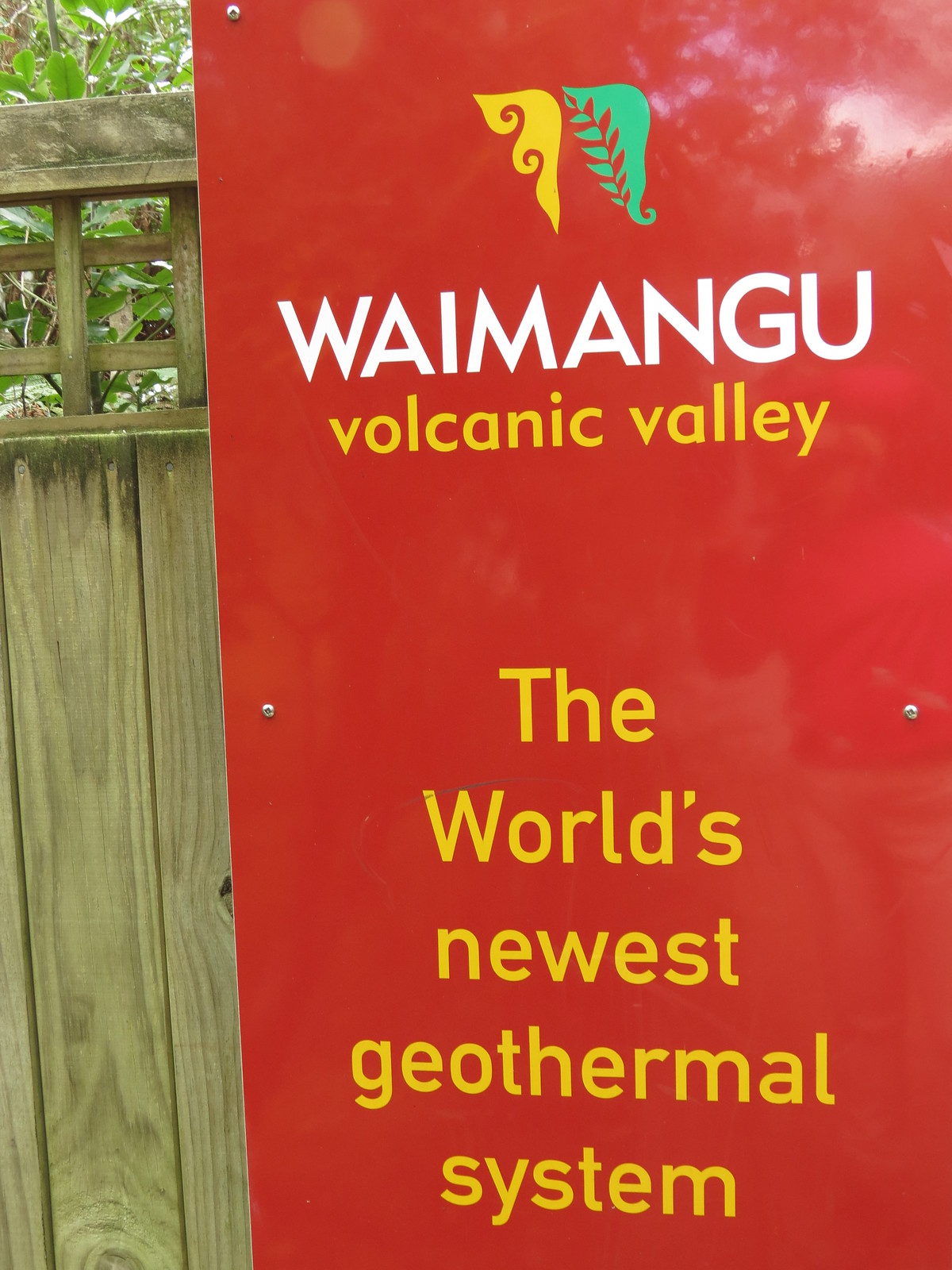This portrait-view image features a vibrant red metal sign bolted to a wooden fence, evident by the visible screws at the top and middle of the sign. The sign's top edge displays a yellow and green leaf image, though the upper part of the sign is slightly cut off. Dominating the sign, central white text proclaims "Waymangu," followed by the message in yellow: "Volcanic Valley," and "The world's newest geothermal system." Behind the fence, glimpses of greenery, trees, and bushes are visible, adding a natural backdrop to the scene. The sturdy wooden fence frames the majority of the red sign, making it a prominent focal point in the image with a natural environment peeking through.